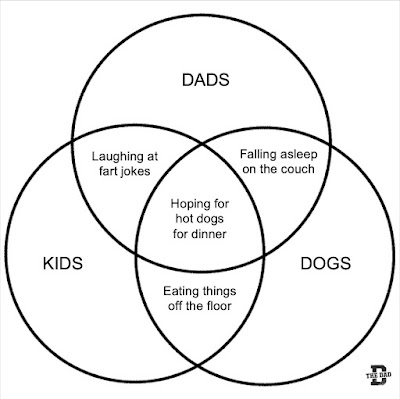The image is a Venn diagram comprising three overlapping circles on a white background with black lines and text in Arial font. The top circle is labeled "Dads" in all caps, the bottom left one "Kids" in all caps, and the bottom right one "Dogs" in all caps. The section where all three circles intersect is labeled "Hoping for Hot Dogs for Dinner." The intersection between Dads and Kids reads "Laughing at Fart Jokes," the intersection between Kids and Dogs reads "Eating Things Off the Floor," and the intersection between Dads and Dogs reads "Falling Asleep on the Couch." A small logo featuring the letter "D" is situated in the bottom right corner of the image.